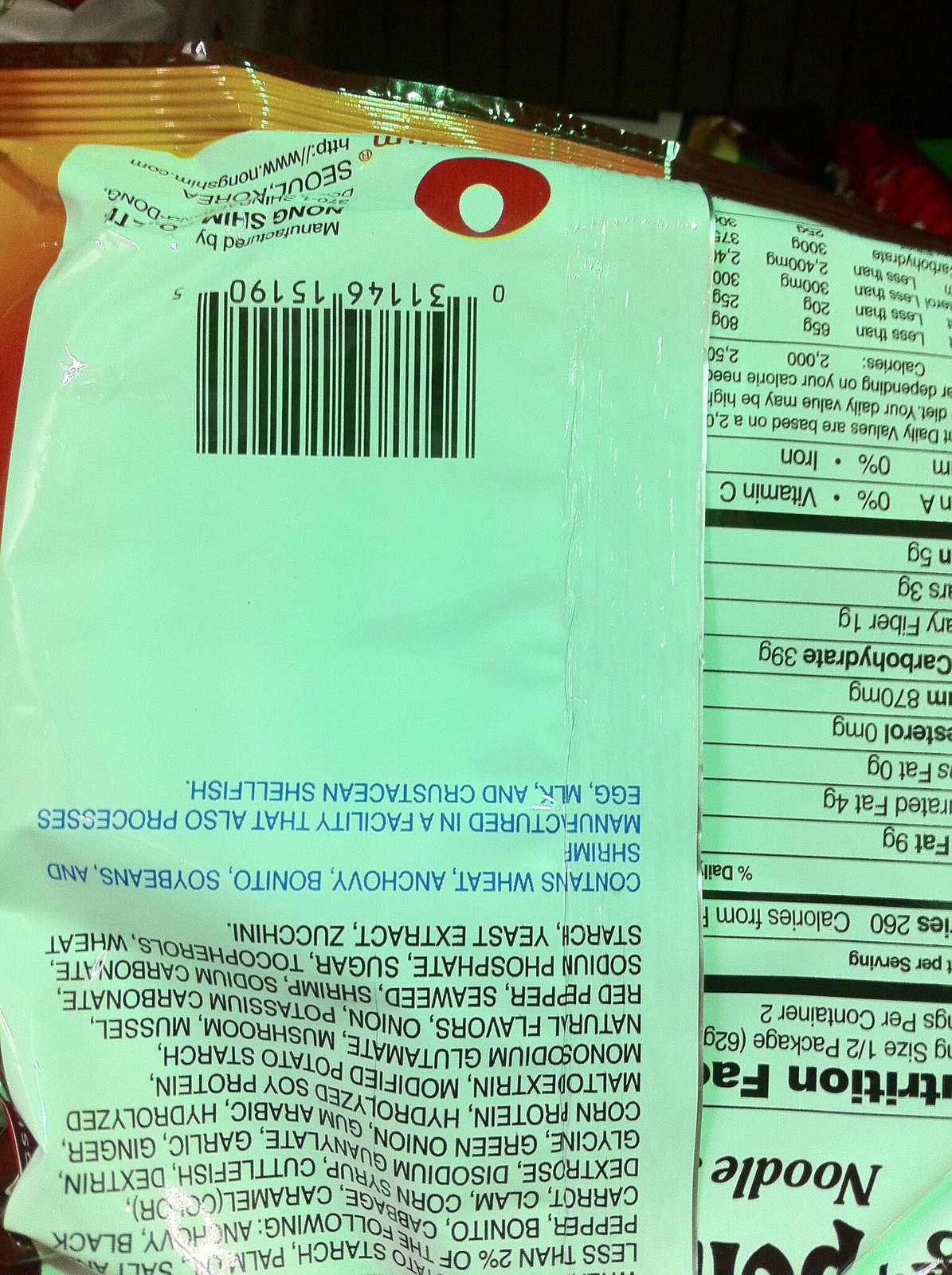This photograph showcases the back of a white food package oriented upside down. In the upper left-hand corner, there is a yellow section with horizontal ridges reminiscent of those found on a bag of chips. At the top of the label, on the left side, there is upside down black writing. Adjacent to the writing, towards the right, there's a red circle with a white circle centered at the bottom. Directly beneath this is an upside down UPC code, centered in a large white space. Below the UPC code, there are four lines of blue text, followed by several lines of black text in all caps, which constitute the ingredient list. On the right side, partly obscured by the flap from the package's front, is the nutrition label. At the top of this label (which appears at the bottom due to the orientation) the word "noodle" is visible.